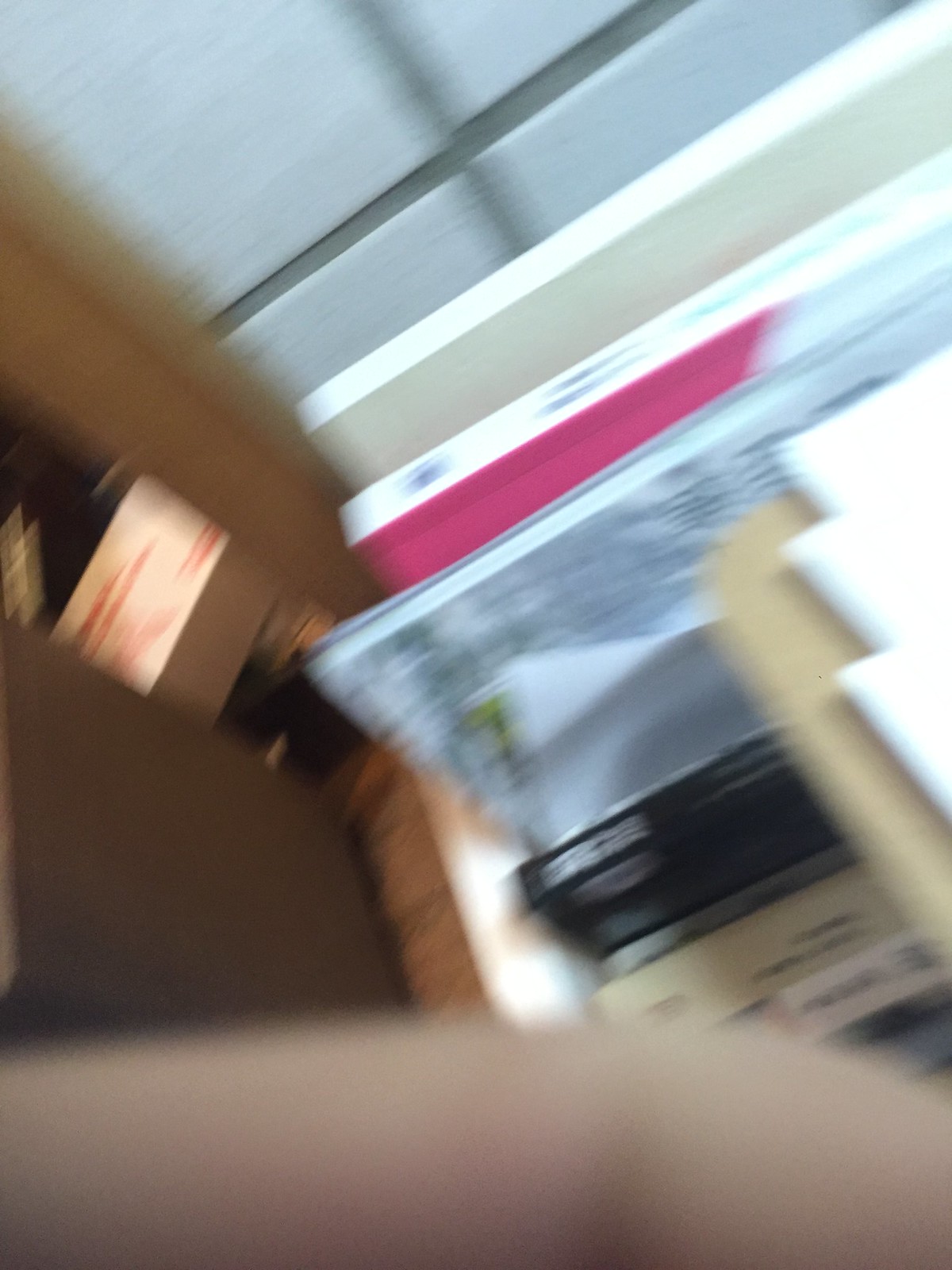The image, captured in portrait mode and turned 90 degrees clockwise, is extremely blurry, making it challenging to discern precise details. At the bottom of the image, a finger, possibly belonging to the person taking the picture and exhibiting light skin tone, partially obscures the view. The interior of a room appears to feature prominently, with a white shelf situated in the middle right of the frame. This shelf is laden with various books of different sizes and colors – notable among them are a book with a white background and pink details, a black book with white writing, a white book with black writing, and a tannish book with black writing. In the top left corner, a rectangular box with red colors and a red logo is visible. There appears to be a brown table with papers on it also positioned near the middle right. Despite these observed elements, the image's overall blurriness makes it difficult to confirm the exact details or full context.